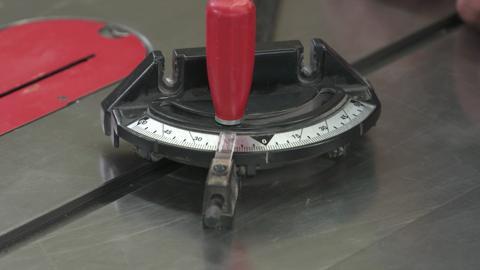The image depicts an intricate component of a table saw, designed for woodworking precision. The central feature is a red, shiny plastic handle that’s part of a measuring device for determining the angle of the saw's cuts. This device is mounted on a semi-circular protractor with degree markings for precise angle measurement, ranging from 0 to 50 degrees. The handle is connected to a black triangular base marked with a zero, indicating perfectly straight cuts. This assembly is securely fitted into a groove on a gray metallic table, which is part of the table saw itself. Surrounding the saw blade, there is a distinct area of red-painted metal, enhancing visibility and safety. Additionally, there are bolts securing parts of the setup to the table. The setup indicates functionality for both left and right angular adjustments, crucial for miter and beveled cuts.